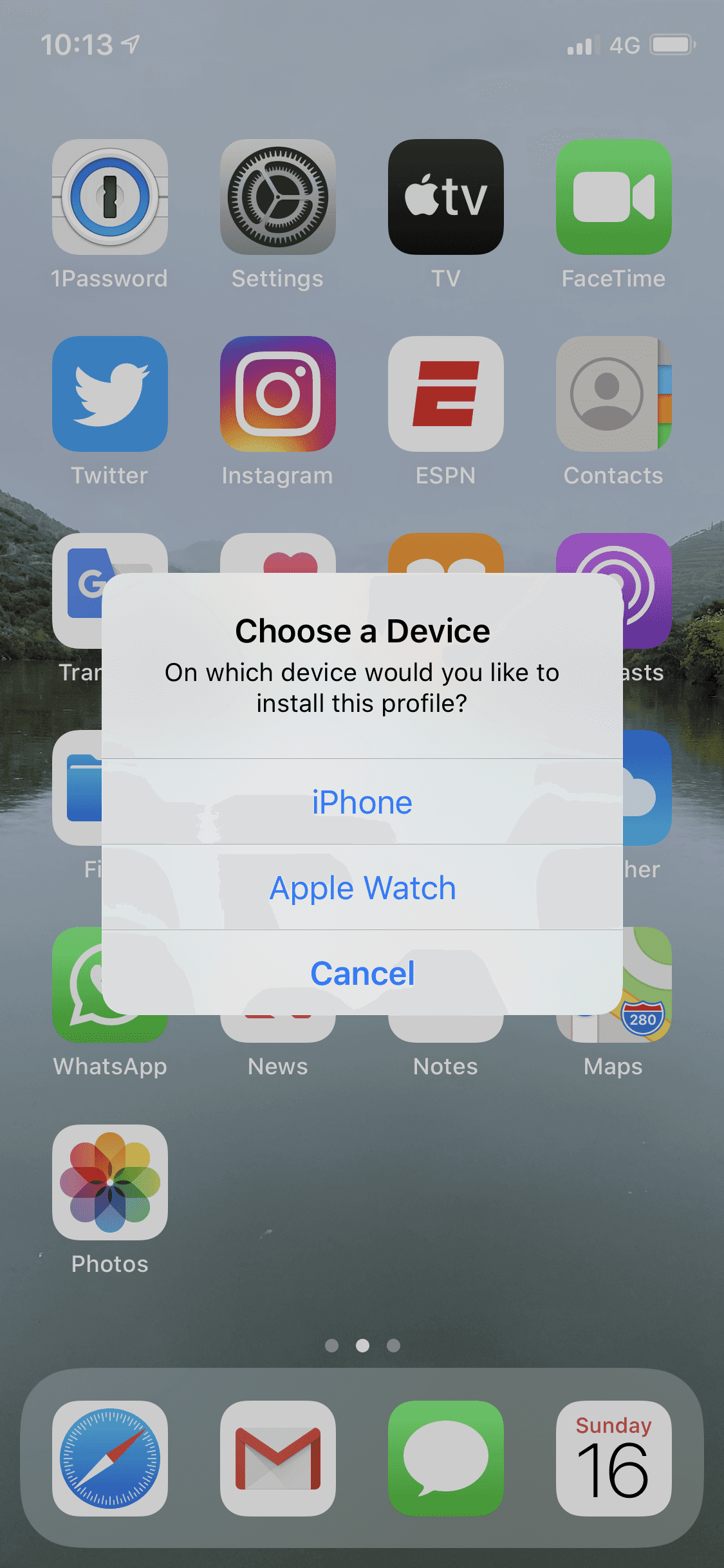The image showcases an iPhone's screen displaying a prompt to choose a device for profile installation. The prompt is positioned at the center of the screen in a white rectangle with the message: "Choose a device. On which device would you like to install this profile?" Below the message, a thin gray line separates two blue text options—"iPhone" and "Apple Watch." At the bottom of the prompt, there's a "Cancel" option.

The home screen, visible behind the prompt, indicates it is 10:13. The top-left corner shows three to four service bars, 4G connectivity, and a full battery. A variety of app icons are arranged on the screen: Password, Settings, Apple TV, FaceTime, Nextdoor, Twitter, Instagram, ESPN, Contacts, Google Translate, Podcasts, Files, Weather, WhatsApp, News, Notes, Maps, and Photos.

The four most recent apps appear at the bottom: a browser, Gmail, a messaging app, and Calendar displaying Sunday the 16th. The wallpaper features a serene lakeside view, with fog and clouds partially obscuring the hills in the background.